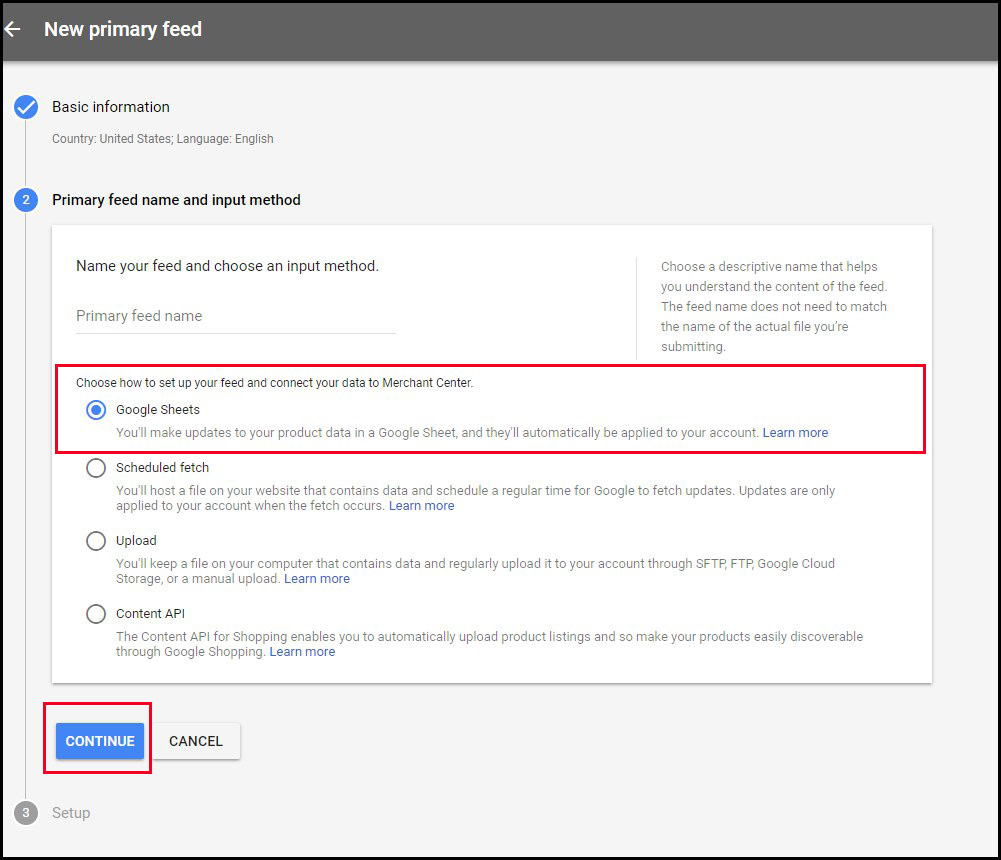Screenshot of a user interface with a heading titled "New Primary Feed" in the top-left corner. The interface displays two lines of text followed by a blue circle, and encompasses a white input box. Within the white box, there are prompts asking to "Name your feed" and to "Choose an input method." The primary feed name input field is shown, along with a red box highlighting the instruction to "Choose how to set up your feed." Options include connecting to Google Sheets, indicated with a blue dot. At the bottom of the interface, there are "Continue" and "Cancel" buttons, with the "Continue" button depicted in a blue square and further emphasized by a red highlight.